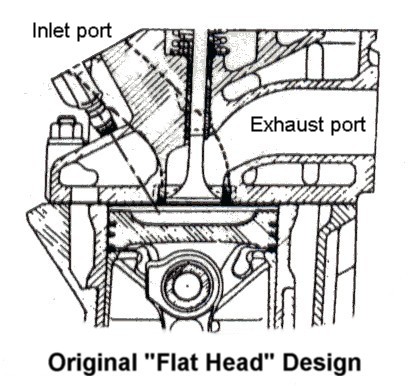The image is a detailed black-and-white mechanical diagram, likely sketched or perhaps digitally generated, focusing on a complex arrangement of parts identifiable as an engine. Key elements include labels such as "Inlet Port" in the upper left corner and "Exhaust Port" to its right. At the bottom, “Original Flathead Design” is prominently displayed, with "Flathead" in quotation marks, suggesting it serves as the title. The diagram features intricate components, including a central tube-like structure, several screw-like elements, and a belt encircling a circular "spinning wheel" mechanism near the bottom. The detailed sketch is characterized by black lines on a white background, indicating an educational tool likely intended for those learning about mechanical trades or engine construction.